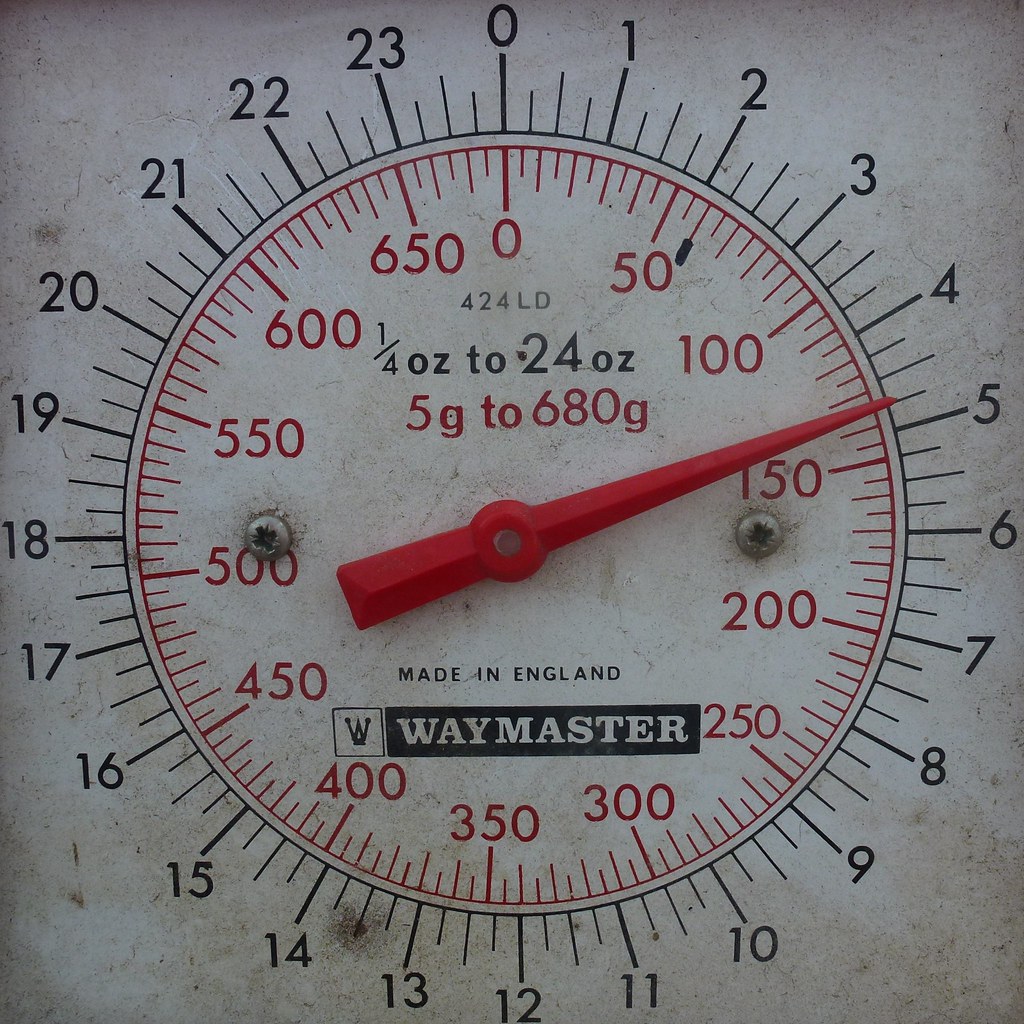The image depicts a precision weighing scale manufactured by Waymaster. Central to the scale is a circular dial with a prominently visible red needle pointing towards the right side of the circle. The dial features two sets of numbers: on the outer ring, black numbers range from 0 to 23 in a clockwise manner, representing ounces, while on the inner ring, red numbers increase in increments of 50, starting from 0 and going up to 680 grams. 

At the top of the dial, black text reads "1 quarter of an ounce to 24 ounces," and beneath it in red is written "5 G's to 680 G grams." The brand name Waymaster is displayed near the bottom in white letters against a black background, alongside the manufacturing detail "Made in England." Small Phillips-headed silver screws are positioned around the dial, securing it in place. The red needle is currently indicating between 100 and 150 grams on the inner red scale and between 4 and 5 ounces on the outer black scale.